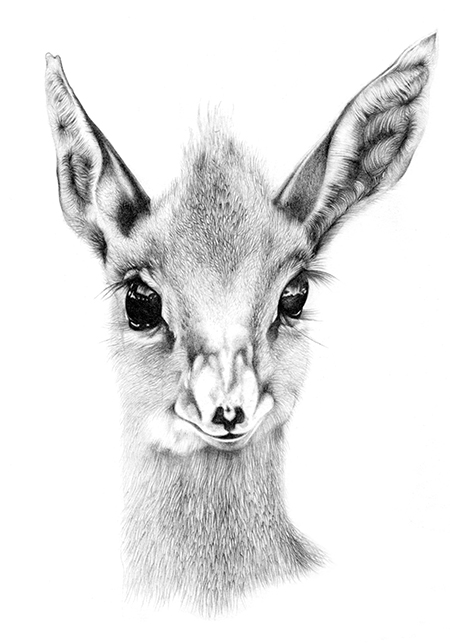The image features an exquisitely detailed, hand-drawn pencil illustration of what appears to be a Dik-Dik's face in black and white. The close-up captures the animal's glossy black eyes, tiny black nose, and small mouth, giving it a slight, almost smiling expression. Its face is covered in thick fur, with a tuft of hair spiking up from the center of its head. The Dik-Dik's long, pointy ears stick out to the sides, adding to its expressive appearance. Surrounding the face, the fur is rendered with intricate detail, notably around the ears and the top of the head, but the neck area fades softly into the plain white background, enhancing the artwork’s natural, delicate quality. This white backdrop allows the features to stand out prominently while creating a seamless blend where the neck dissolves at the bottom. The overall effect is that of a finely crafted, realistic portrait that could easily be mistaken for a photograph.